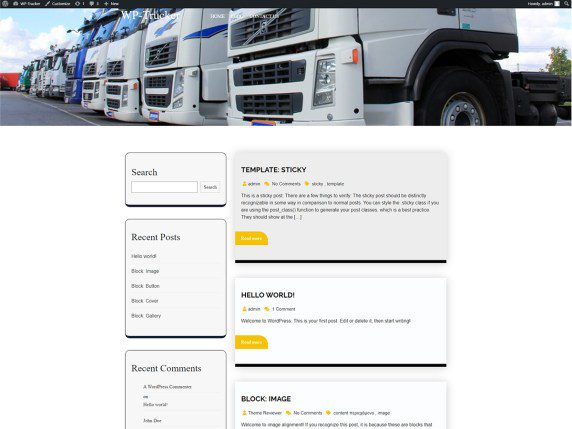At the top of the image, there's a front-facing view of a long row of semi-truck cabs. These trucks have no trailers attached, showcasing their flat front ends prominently. The trucks are mostly white, each featuring distinct grilles and tall vertical headlights, with the exception of a single blue truck in the center. There are about 10 to 12 trucks in this row.

Below this image, there's an interface showing an empty search bar. To the left, there is a section labeled "Recent Posts," and underneath that, another labeled "Recent Comments." To the right, the bold black text reads "Template" and "Sticky." Further down, there's an informational area with the bold black text "Hello World," followed by an exclamation point. Lastly, there is a section titled "BLOCK: Image" in uppercase letters. This section contains three tiny sub-areas separated by yellow circles, with the center one labeled "No Comments."